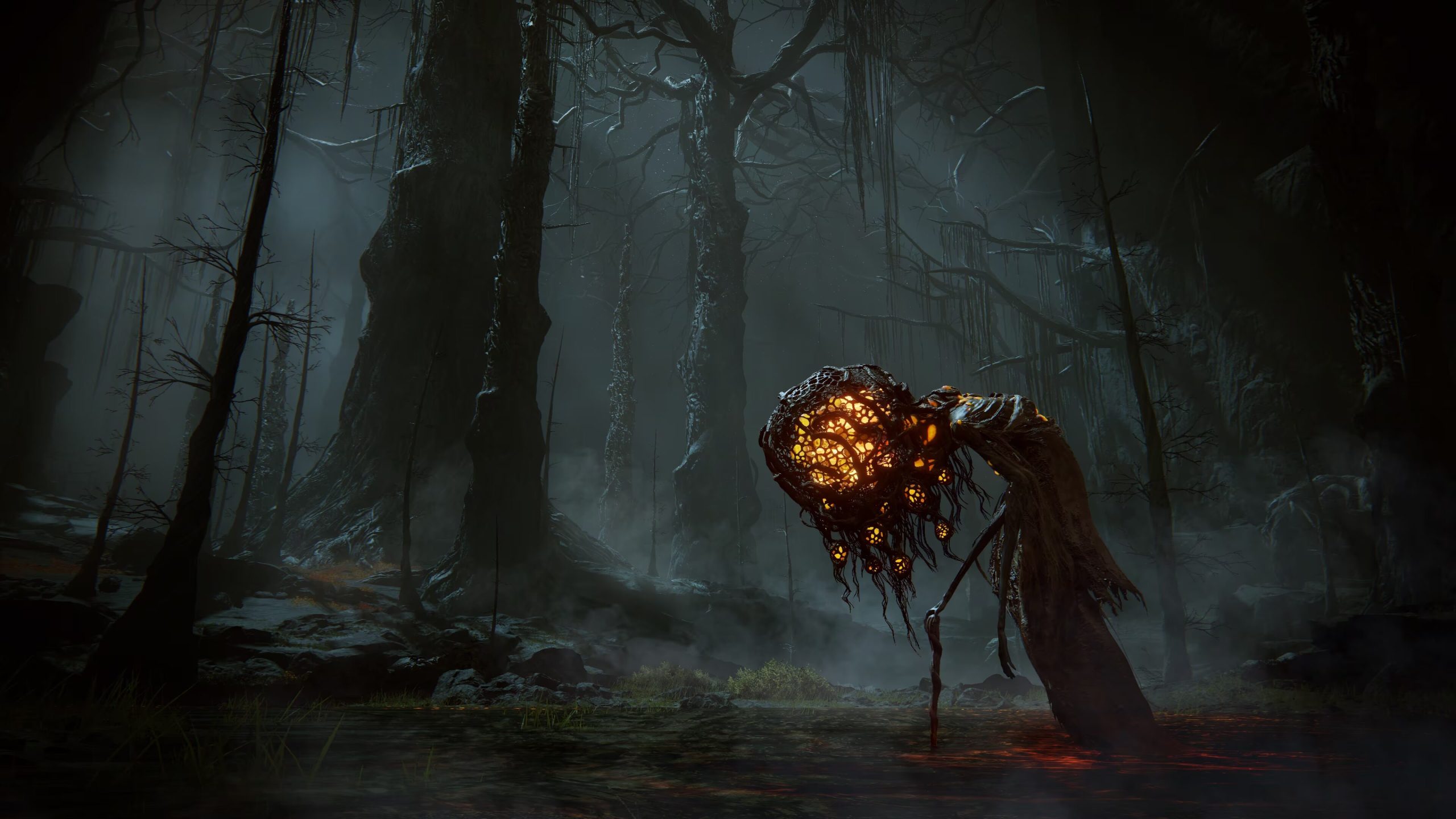In the dim and eerie forest scene, shrouded in darkness and smoke, stands a disturbing yet enigmatic figure that commands attention. The tall, blackened trees extend their nearly bare limbs, some adorned with hanging moss, contributing to the overall gloomy atmosphere. On the forest floor, scattered and lifeless foliage peeks through the obscurity.

Illuminated slightly to the right of the center, a peculiar, humanoid figure captivates the eye. Resembling an old person bent over to the left, this figure emanates an unsettling glow from its head, which appears to be a bright orange orb cloaked in netting or hair-like tendrils. The light extends through skeletal, spindly limbs, which give the impression of two bony hands clasping a stick for support. The figure is dressed in tattered, gray attire reminiscent of an ancient, possibly 1700s military uniform.

Beneath this spectral entity, the ground glows faintly red, adding to the otherworldly and mystical aura. The combination of the skeletal features and the odd light patterns suggest an artistic creation rather than a living being, evoking a sense of haunting mystique perfect for a scene out of a horror narrative.